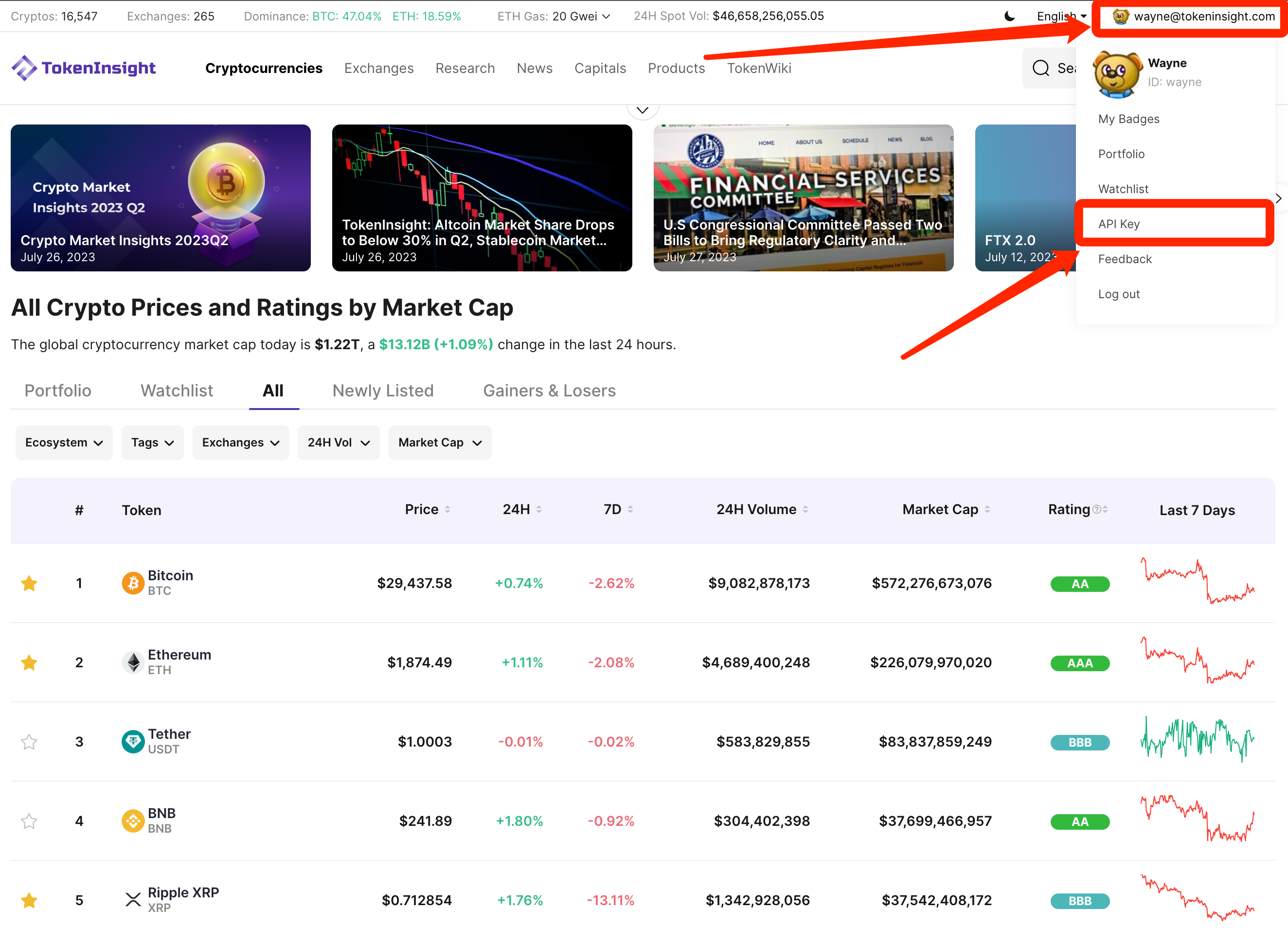This cropped screenshot from the Token Insight webpage provides a clear and detailed guide for accessing the API Key section. The interface features a clean white background with the Token Insight logo prominently displayed on the left. In the top right corner, the user login area shows a profile picture and the email address of the logged-in user, highlighted by a red box and an arrow for emphasis. Below this, a pop-up box appears, reiterating the user's profile photo and screen name. Within this pop-up, there are six selectable categories: "My Badges," "Portfolio," "Watchlist," and "API Key," with "API Key" specifically highlighted by another red box and arrow. The visual cues guide users through the steps: first, clicking on their login information and then selecting the "API Key" option.